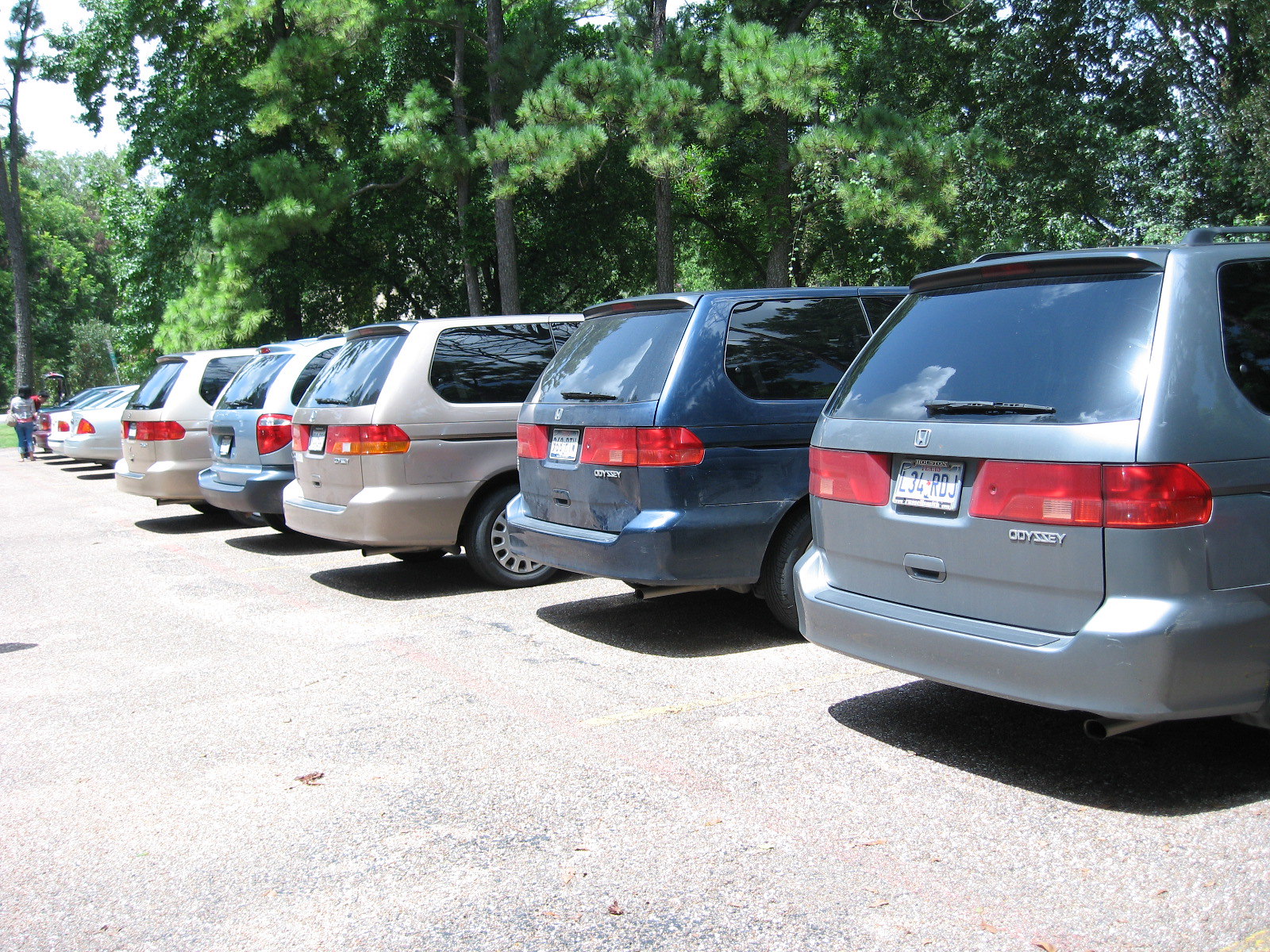In the foreground of the image, several vans and cars are parked in a faded asphalt parking lot bordered by a forest and park area. Notably, there are three Honda Odysseys parked side by side, distinguished by their colors—gray, blue, and tan—all seemingly from the same model year. The lot shows faint white parking lines, indicating designated spaces. The bright morning sunlight casts distinct shadows from the vehicles onto the pavement. The top portions of the image reveal brown tree trunks and lush green foliage, including needle-like leaves of coniferous trees, indicating a forested background. A person can be seen standing on the far left side. In the distance, additional cars and possible people are visible.